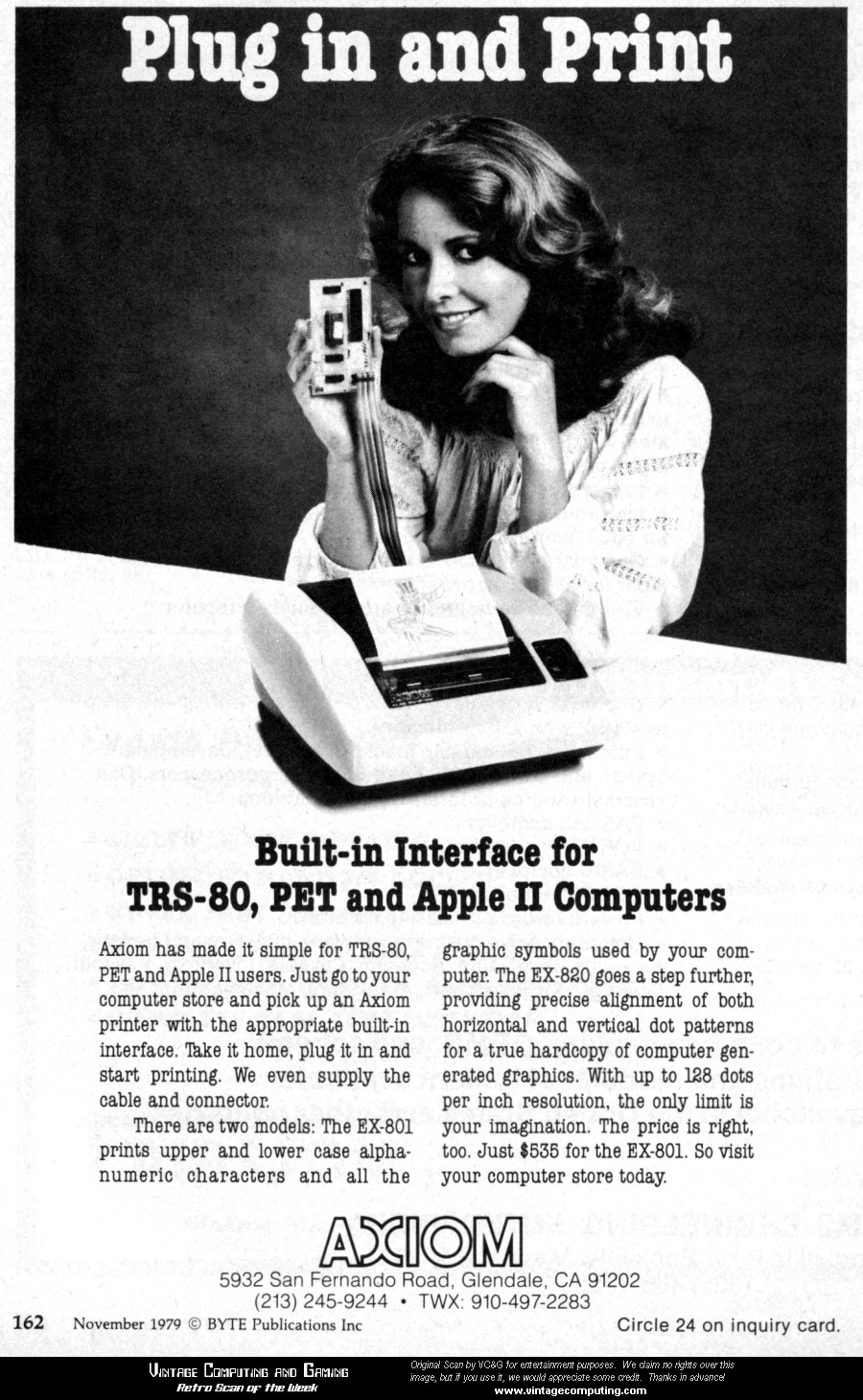This vertically rectangular black-and-white advertisement from November 1979 promotes an early printing machine. The layout features a two-part background: the top half in black and the bottom in off-white. At the top, the white text reads "Plug in and print." Below this, a young woman with wavy, dark hair smiles at the camera. She is dressed in a white blouse, resting her elbows on a tabletop while holding a rectangular device that appears to be a camera or similar contraption, with a strip of film or printed paper emerging from it. On the table in front of her is an early-model white printer producing a sheet of paper. The advertisement highlights a "built-in interface for TRS-80, PET, and Apple II computers" in black text beneath the image, followed by two descriptive paragraphs. At the bottom, within a black border, the company's name, "Axiom," is prominently displayed, along with their address and phone number.